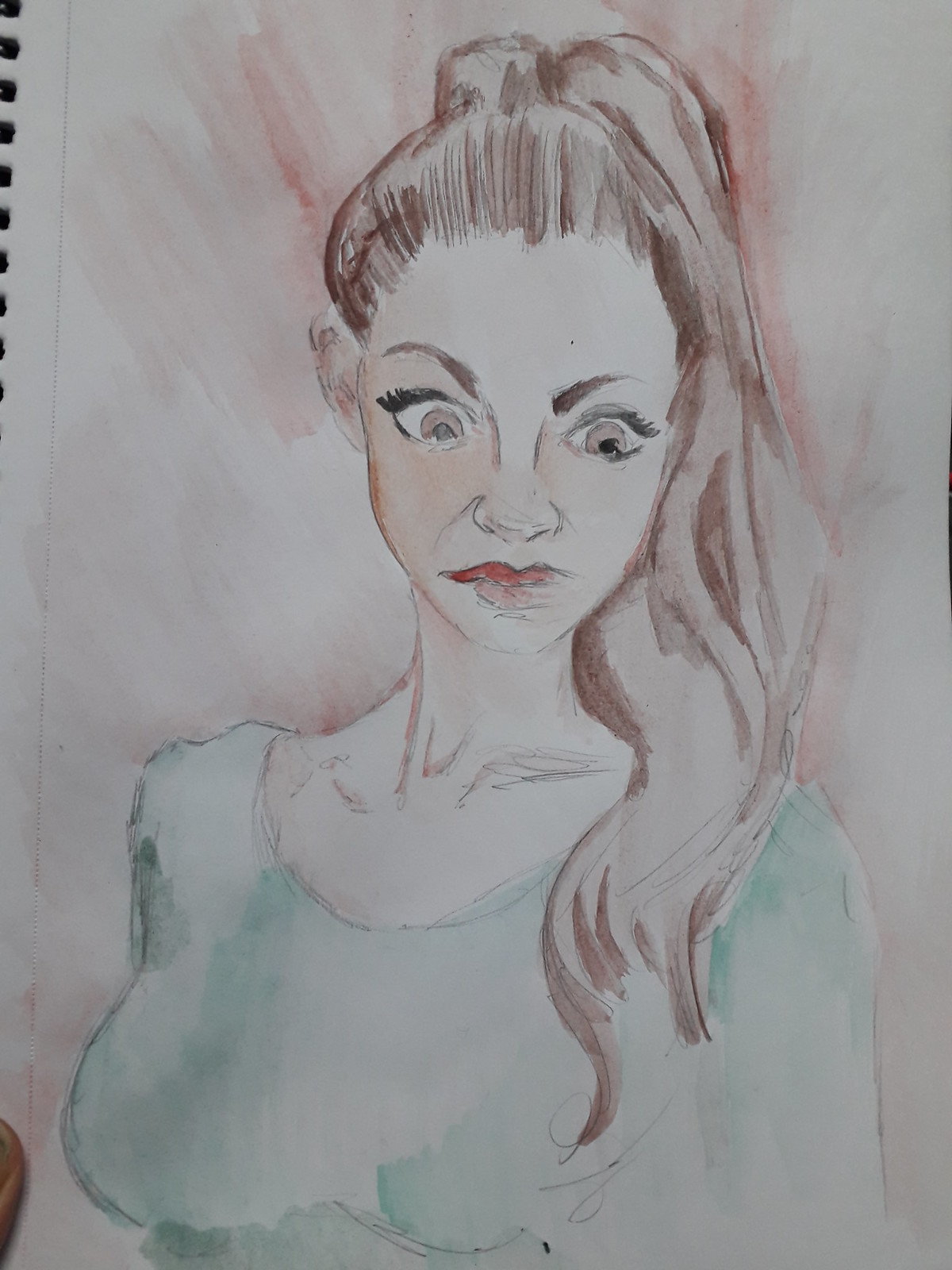This watercolor painting on white paper, depicted in a sketchbook with visible binding on the left, features a woman with an intense, almost psychotic expression. Her long brown hair is pulled into a high ponytail that cascades over her left shoulder and down to the tops of her breasts. She is wearing a light blue top that highlights her sizable bust against her narrow frame. Her elongated neck and defined clavicle, along with the detailed shading, add depth to her appearance.

The woman's face is striking and angular, framed by dark, arched eyebrows and long black eyelashes. She has wide, brown eyes with one noticeably dilated pupil, contributing to her unsettling stare. Her lips are full and red, though asymmetrically represented, adding to the distorted, dramatic effect. Her cheeks have a slight blush, and there is a reddish-brown aura in the background, enhancing the sense of intensity. The detailed depiction of her neck muscles further accentuates the tension in her pose.